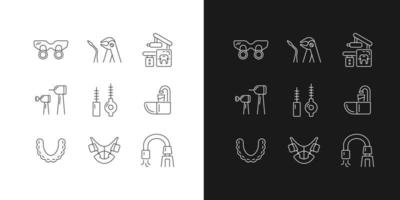The image consists of two adjacent squares, each containing nine small, black-and-white, high-contrast icons arranged in a 3x3 grid. The left square features black icons on a white background, while the right square showcases white icons on a black background, with each icon mirrored in both squares. The top-left icon resembles a car or mask, and the top-middle icon is a tool or wrench. The top-right icon appears to depict equipment related to dental work. In the second row, the left icon resembles a dental drill, the middle icon is likely a dental bit, and the right icon looks like a sink from a dental office. The bottom-left icon seems to be a retainer, the middle icon is linear, and the bottom-right icon looks like a suction device used in dental practices.